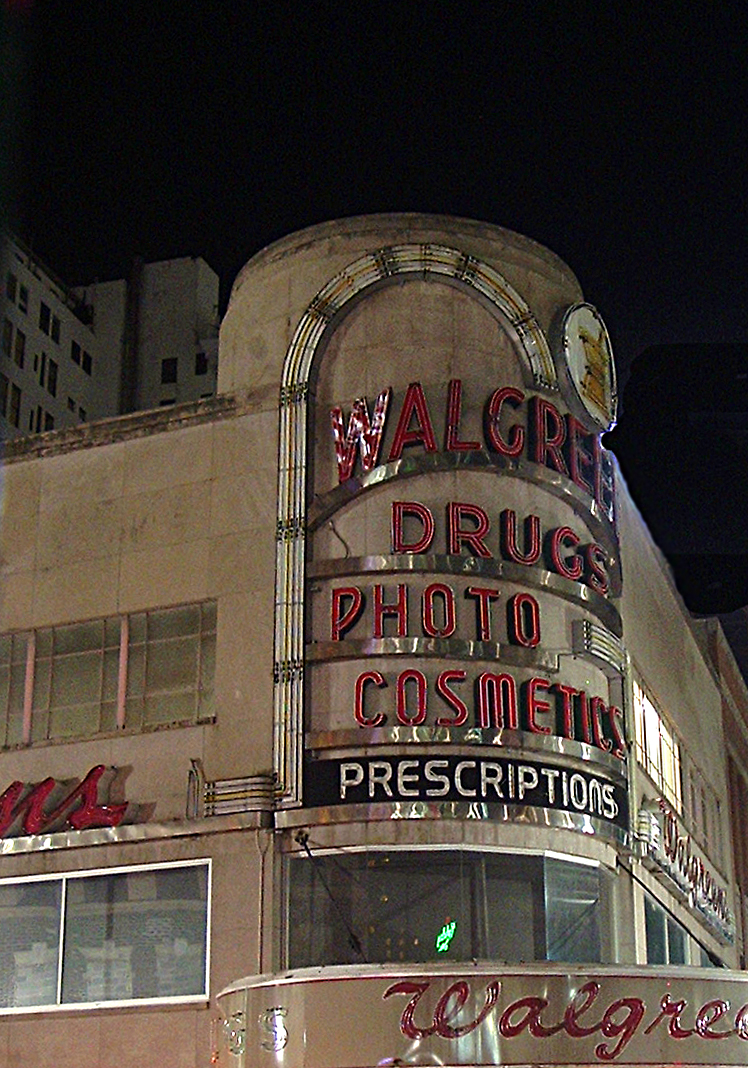This photograph showcases a striking Walgreens building adorned with vintage-style signage reminiscent of the 1950s. The structure appears to be constructed from smooth cement, resembling stone tiles, though not quite marble. The façade is characterized by its old-school windows, reinforced with straight bars, and intricate metalwork above them. The iconic Walgreens signage features a frame that likely illuminates when the store is open. The words "Walgreens," "drugs," "photo," "cosmetics," and "prescriptions" are emblazoned in bright metallic red, with an additional "prescriptions" label beneath in silver letters on a black background. The Walgreens name is prominently displayed multiple times—centrally and on both flanking sides. Numerous windows punctuate the building, some visible and some obscured. The scene is set at nighttime, with the glow of city lights adding drama, and a towering building looms to the left, adding to the urban landscape.